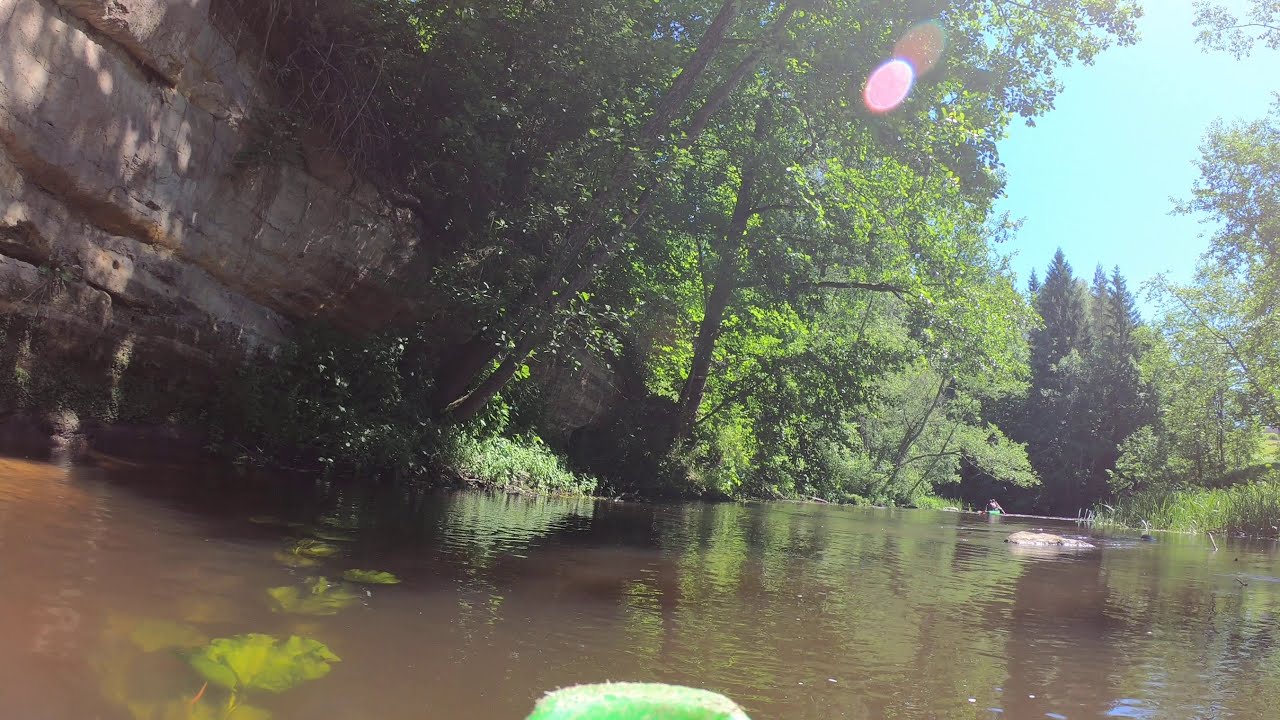This photograph captures a scenic river view from near its water surface. The predominantly brown water, dotted with green-leaved plants, reflects the clear blue sky above, which is bathed in warm sunlight. On the left shore, towering rocky walls, colored brown and accentuated with green moss, create a stunning natural border. The riverbanks are lined with lush trees on both sides, adding to the verdant scenery. Further into the river, a green boat manned by several people is visible. Interestingly, there appears to be an unidentified animal, potentially a crocodile or hippo, partially submerged in the water. The overall atmosphere is serene and bright, indicative of a warm, sunny day.